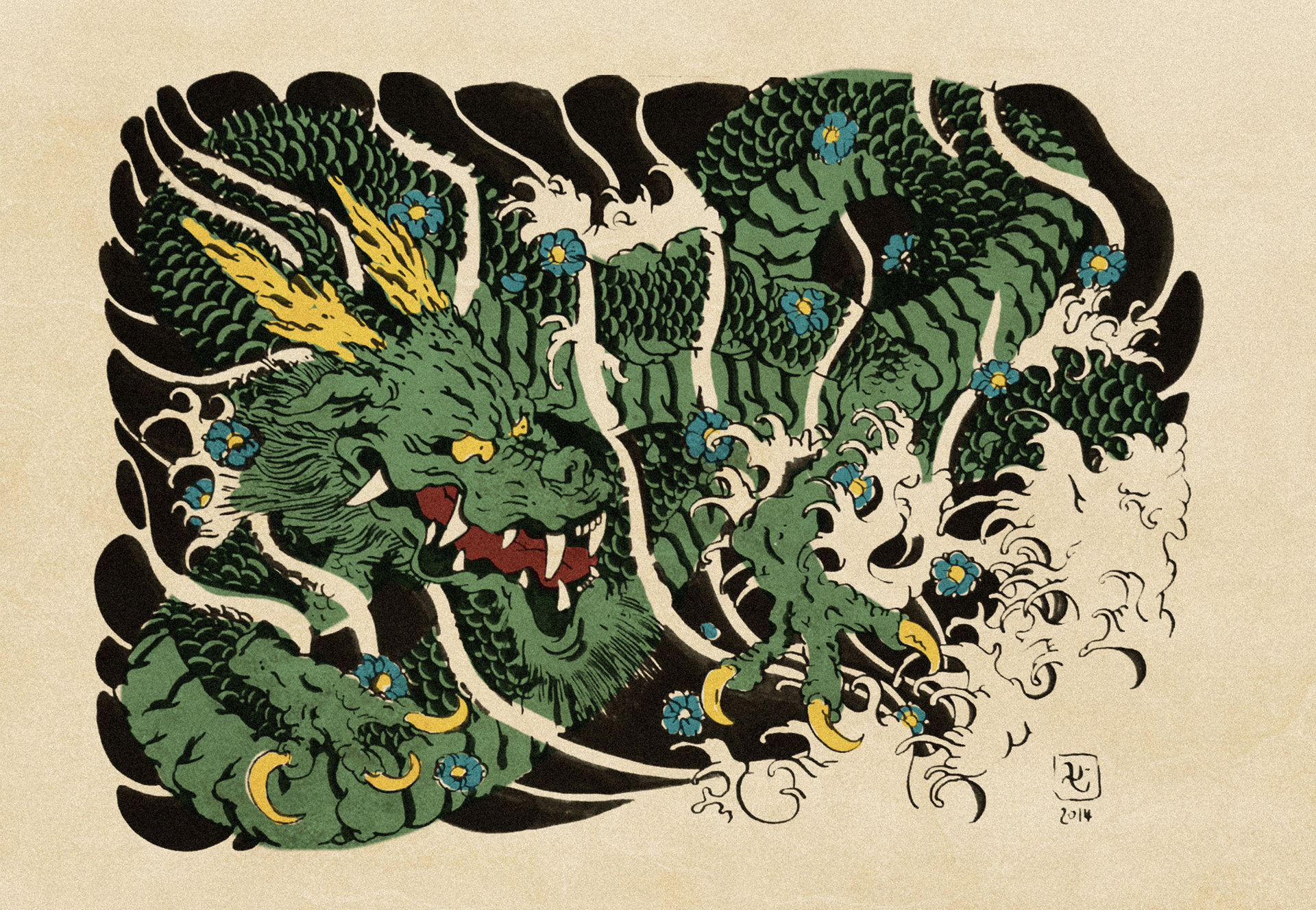This detailed artwork showcases a Japanese-style green dragon with an array of vivid features: aggressive yellow eyes, yellow talons, and prominent yellow horns protruding from its head as if made of flames. The dragon's broad snout displays numerous long, sharp fangs spaced widely apart above a dark reddish-brown, elongated tongue. Its sinuous body, covered in menacing black scales, curves gracefully from left to right and then back to the left again. 

Striking against a black background, the dragon is set on manila-colored or whitish-beige textured paper. The dragon is adorned with teal and blue-hued flowers, each with a yellow center, symbolizing traditional Japanese designs. Surrounding the dragon are intricately drawn white patterns reminiscent of water splashes or clouds, adding a dynamic and ethereal dimension to the artwork.

In the lower right corner, there is a red-inked artist’s seal featuring a single black character along with the date "2014," marking the piece's creation. This meticulous fusion of traditional Japanese tattoo motifs with modern artistic techniques embodies the timeless essence of mythical imagery.